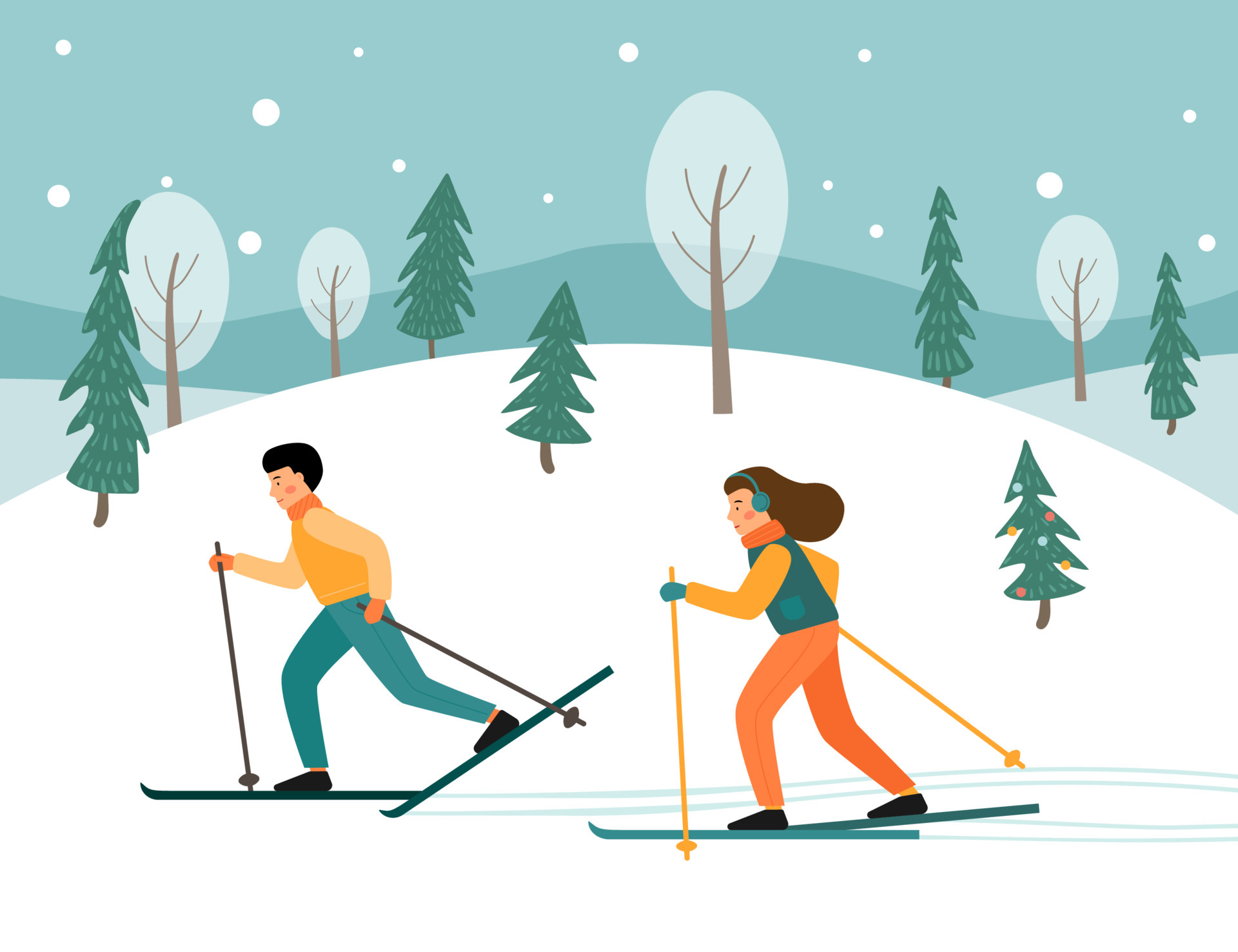The digitally composed, cartoon-style image features a winter scene where a man and a woman are skiing from right to left on a snowy hill. The sky is light blue, dotted with white circles depicting falling snow. A darker blue, curving mountain forms the backdrop, interspersed with various trees that have straight brown trunks and green triangular clusters for foliage, as well as leafless, snow-covered trees.

In the foreground, the snow-covered hill extends across the scene, dotted with these distinctive trees. The man, positioned on the left, has short brown hair and is adorned in a light yellow jacket with a long-sleeved shirt underneath, blue pants, black shoes, and dark blue skis. He also wears an orange scarf and gloves. The woman, skiing slightly behind and to the right, has long brown hair flowing behind her, dressed in a blue jacket with yellow sleeves, an orange scarf, blue gloves, orange pants, black shoes, and lighter blue skis. She also sports blue earmuffs. The overall setting, reminiscent of a folksy, Grandma Moses art style, captures the essence of a quaint winter day.